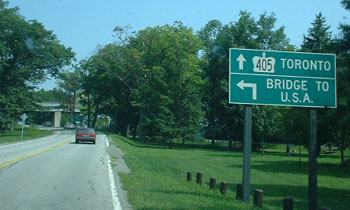The image depicts a bright and sunny day with a vivid blue sky, showcasing a straight section of a road that leads to a leftward curve beneath an overpass. Framing the road are large trees with lush green leaves, positioned on both the left and right sides. The road itself, likely asphalt or concrete, features prominent yellow lines in the middle and white lines on the sides. A single, darker-colored sedan is visible in the distance, making its way toward the curve. On the right side of the image, there is a well-maintained grassy slope that descends into a larger green area. Prominently displayed is a large, green highway sign with a double post: the top part directs traffic straight ahead to "405 Toronto" with a distinct crown-like emblem surrounding it, and below it, an arrow pointing left indicating "Bridge to USA." This suggests the image is taken near an international border, potentially providing routes towards Toronto and a bridge crossing into the United States.